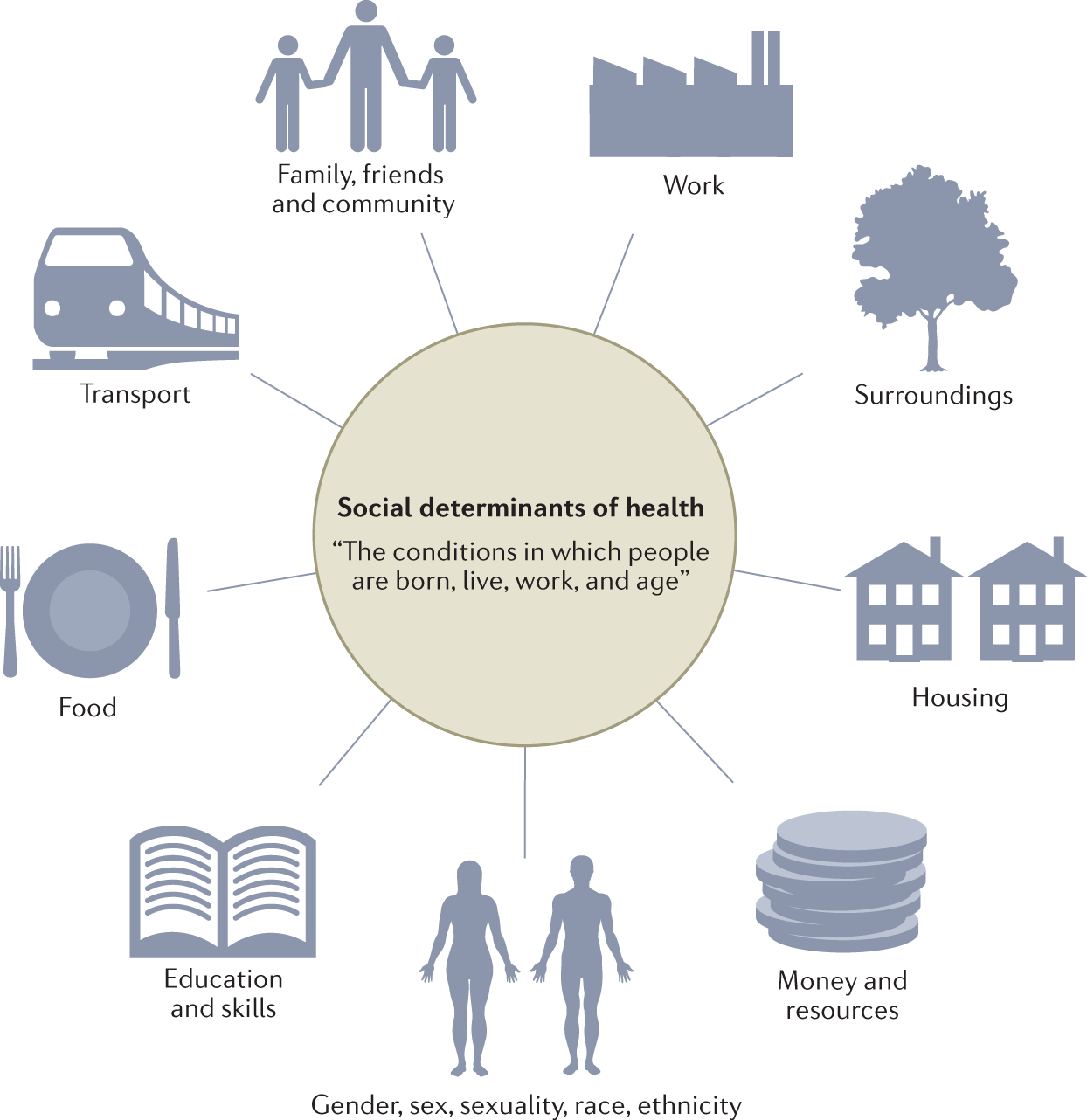The image is an informational graphic or diagram illustrating the Social Determinants of Health, set on a white background. At the center of the diagram is a light gray circle containing the text, "Social Determinants of Health: The conditions in which people are born, live, work, and age." Radiating out from this central circle are lines connecting to various icons and labels that represent different social determinants. 

Starting from the top left and moving clockwise, the icons and their corresponding labels are as follows:

1. **Family, Friends, and Community** - represented by three silhouetted figures holding hands.
2. **Work** - depicted by the silhouette of an industrial building.
3. **Surroundings** - shown with the silhouette of a tree.
4. **Housing** - illustrated by two house silhouettes.
5. **Money and Resources** - symbolized by a stack of coins.
6. **Gender, Sex, Sexuality, Race, and Ethnicity** - indicated by the silhouettes of a man and a woman.
7. **Education and Skills** - symbolized by a book icon.
8. **Food** - represented by a plate and utensils.
9. **Transport** - shown with the silhouette of a train.

All the icons are simple line drawings or silhouettes, and they are arranged in a circular layout around the central circle, highlighting the comprehensive nature of factors impacting health.